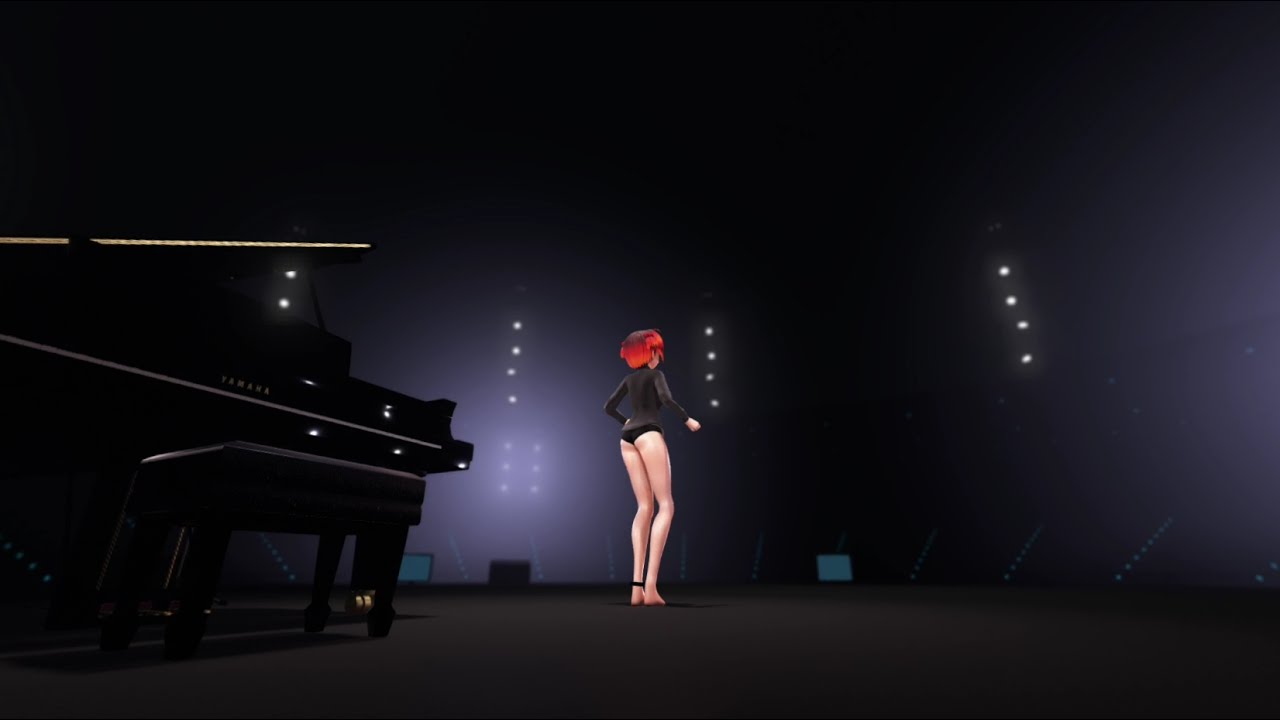This AI-generated image depicts a striking scene on a dimly lit stage. In the center, a woman with short red hair stands facing the audience, her back to the camera. She is wearing a black long-sleeved top and black underwear, giving an impression of casual attire or rehearsal wear. Her left ankle is adorned with a black light, adding a curious detail to her outfit. The stage's background is entirely black, contrasted by white spotlights on the wall that cast a cool glow across the scene. To the left side of the stage, there's a black grand piano with a gold trim and a bench in front of it. Above the piano, a thin yellow line can be seen. The floor is dark black, and along its edge, monitors with blue-gray screens are visible. The audience is positioned to the right side of the image, suggesting an imminent performance or a rehearsal setting. The overall atmosphere is moody and intense, highlighting the anticipation and preparation before a concert.